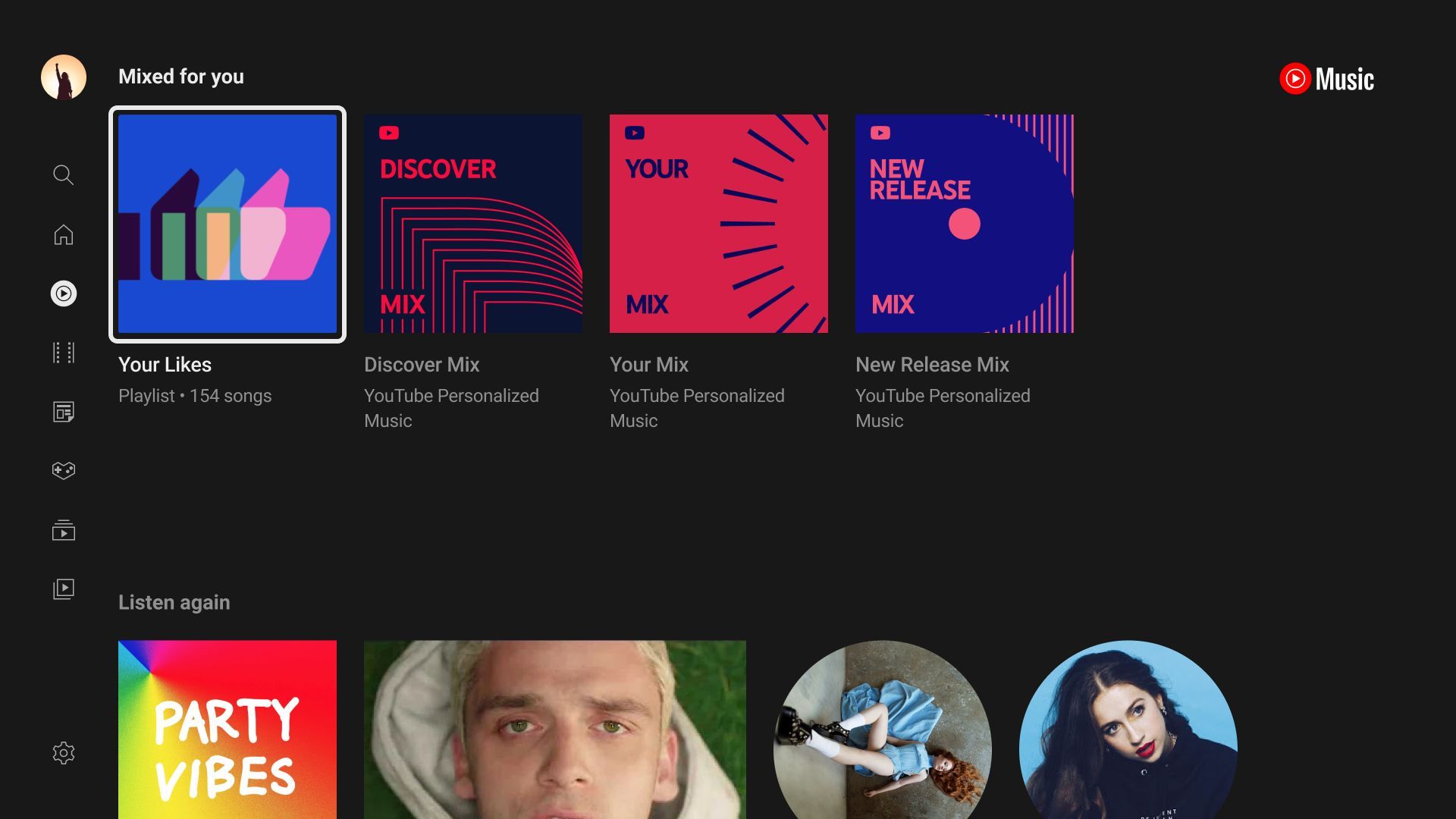The screenshot depicts a desktop view of a YouTube Music interface, though the image is cropped. In the top-left corner, there is a user avatar showing a person with their arm raised. Below this avatar, various icons are lined up vertically: a magnifying glass (search), a house (home), a circular play button, an old-fashioned film reel, a folded piece of paper with data, a heart resembling a game controller (with additional icons beside it), two distinct play buttons with different arrangements of squares behind them, and a cogwheel (settings).

Continuing towards the center, the screen displays a section titled "Mixed For You." It features an album cover with multiple colorful thumbs-up icons, labeled "Your Likes Playlist" consisting of 154 songs. Below that, there is a "Discover Mix" section with red and dark blue tones, indicating a personalized music mix. Adjacent to it is another mix labeled "Your Mix" in red and blue hues, with an image of lines emanating from a sun and a blue CD or LP with pink text and lines.

Further down, a "New Release Mix" section is highlighted, also personalized by YouTube Music, followed by the platform’s logo to the right. At the bottom, the "Listen Again" section appears with a "Party Vibes" banner in rainbow colors, featuring images of musical artists. The first artist is a Caucasian male with green eyes and bleach-blond hair, lying down. The second is a woman in a pale blue, flowing swimsuit-like outfit, with coppery brown hair, white socks, and black platform shoes, shown horizontally. The final artist is a woman with black hair, dark eyes, red lips, and a black sweater, posed with her head tilted to the side. These images presumably represent artists the user has previously listened to on YouTube Music.